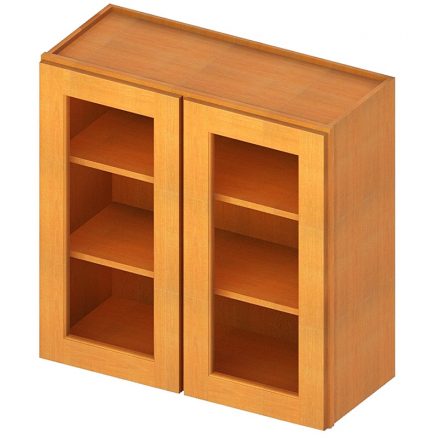The image depicts a small, square-shaped wooden cabinet with a plain, box-like appearance and a beveled edge along the top. Crafted from light wood grain, the cabinet is shown in a top-down isometric view against a white background, with light coming from the upper right, casting shadows inside. The front features two shaker-style doors with glass cutouts, revealing two interior shelves. The doors are stained in a lighter shade than the exterior of the cabinet, emphasizing the simple yet elegant design. The cabinet's orientation is diagonal to the viewer, giving a clear perspective of its subtle details, suggesting it could be an illustration for a catalog.